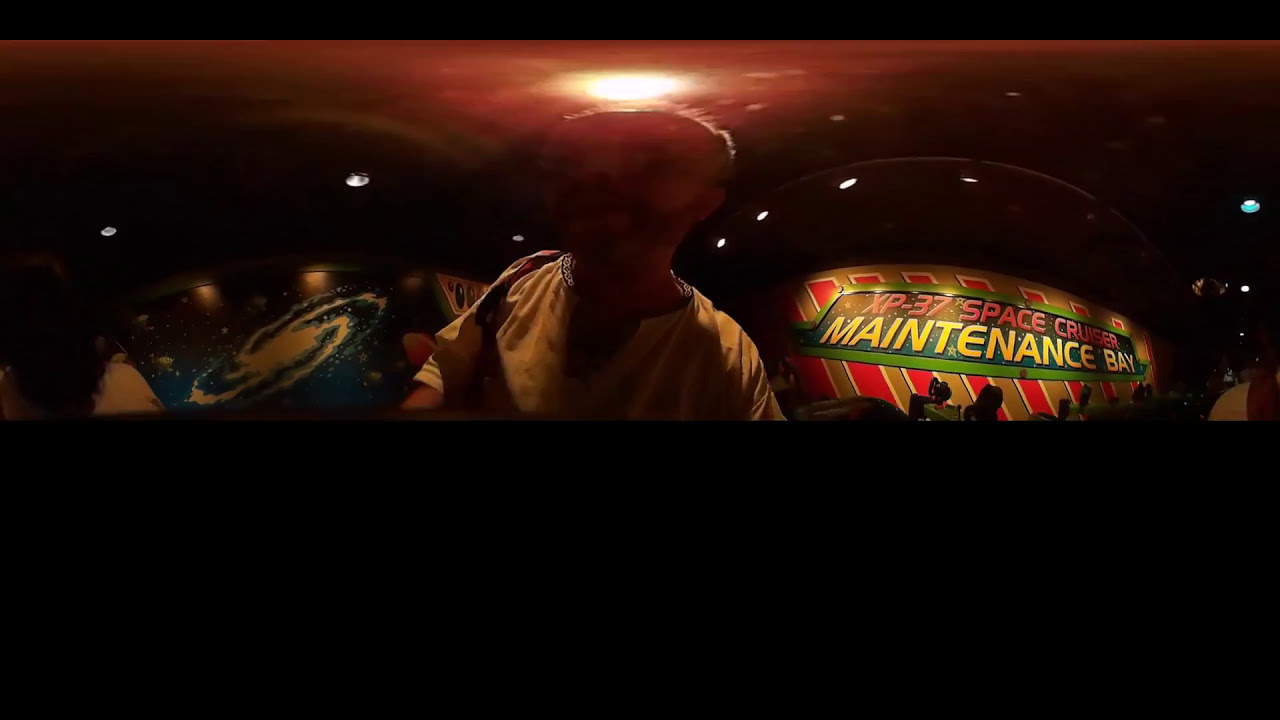This photograph, with a panoramic wide-angle view, captures an indoor nightclub or arcade setting under dim, dramatic lighting. The center of the image features the silhouette of a man, albeit his ethnic background isn't discernible. He is attired in a gray shirt, accentuated by a blue lanyard. A yellow overhead light casts a reddish hue, creating a stark contrast against the surrounding darkness, leaving the man's face obscure.

To the man's left, partially illuminated, is a vivid graphic of a galaxy set against a black sky, presenting a swirling cosmic display. To the right, another point of interest emerges: a sign with red and gold stripes and a green border proclaiming "XP-37 Space Cruiser Maintenance Bay," hinting at a sci-fi theme likely tied to the venue. Silhouetted equipment rests before this sign, adding to the immersive ambiance.

The composition is bordered by a solid black band at both the top and the bottom, framing the central elements in an almost cinematic fashion. Dark lights sporadically punctuate the space, emphasizing the photograph's overall moody and mysterious atmosphere.